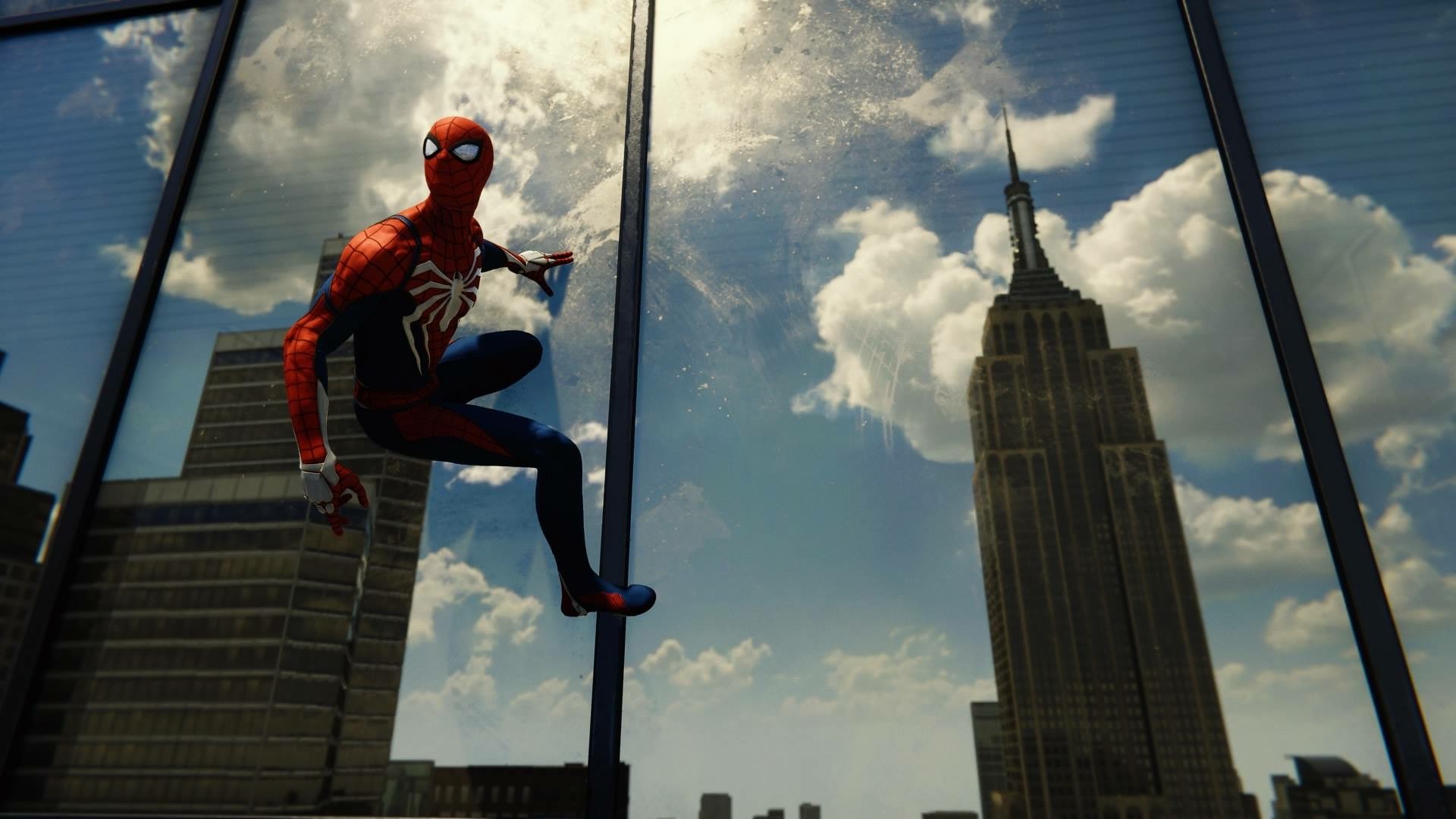In this striking image, Spider-Man clings to a glass window on a towering skyscraper, evoking a scene from the iconic movie. The window reflects a beautifully clear, sunny day with a vibrant blue sky and scattered white clouds. To the right of the reflective glass, there's a glimpse of another tall, gray building crowned with a spire, while on the left, two more imposing structures stand tall. Spider-Man, donned in his classic red suit adorned with the white spider emblem and blue lower half, appears poised for action. His right hand is firmly pressed against the glass, and he seems to be preparing for his next leap. The reflective cityscape adds depth to the photograph, with Spider-Man’s dynamic pose capturing a moment frozen in time, reflecting his readiness and agility.